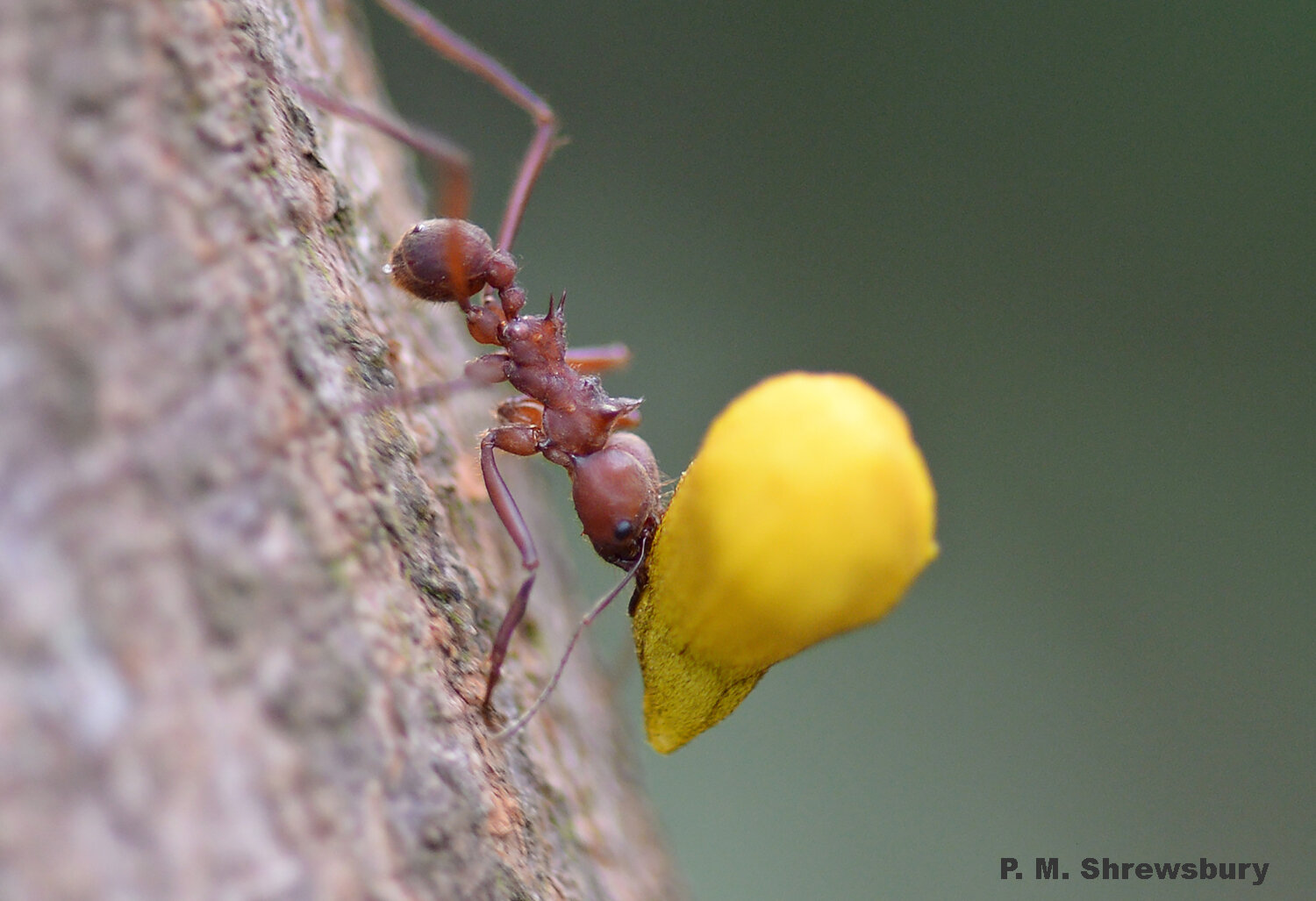This detailed close-up photograph captures a reddish-brown ant, notably vivid in its intricate anatomy, as it descends diagonally down a tree bark or rocky surface. The ant, with its six legs and distinguished body segments—the head, thorax, and abdomen—strikingly contrasts the blurred green and gray background, emphasizing its focus. In its powerful mandibles, it carries a large, yellow kernel or piece of vegetation, significantly larger than its own body. The ant's impressive strength is on full display, highlighting its ability to carry loads much heavier than itself. The photograph, signed P.M. Shrewsbury, underscores the remarkable detail and strength of this small yet mighty insect.